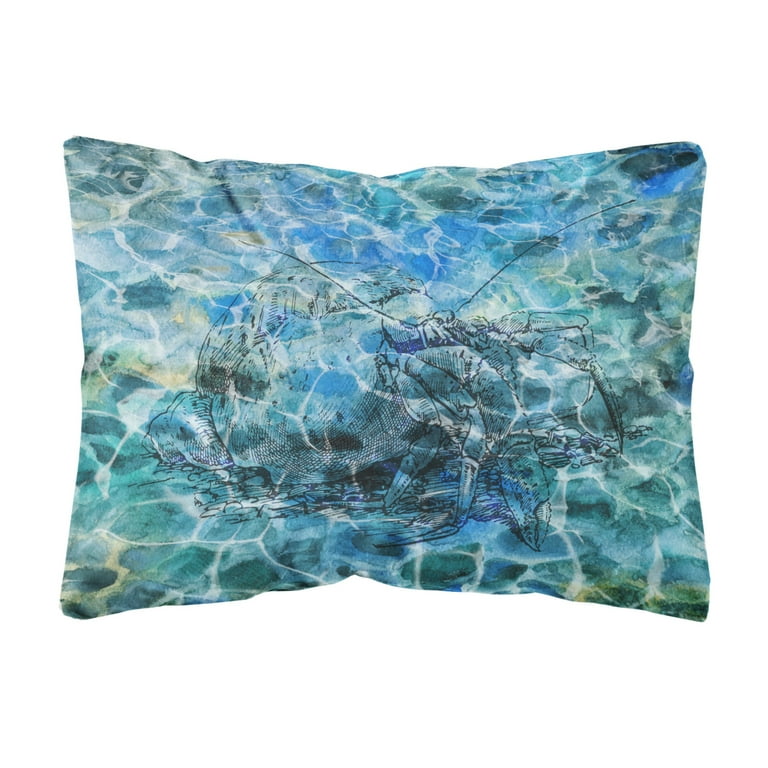The image is a detailed product photo of a rectangular pillow adorned with a complex, ocean-inspired design. Predominantly in blues, greens, and turquoise, the pillow features a pattern that resembles a turtle shell. At the center of this pattern is an intricately sketched image, likely of a crab or a similar sea creature, with distinguishable claws and antennae. This central figure is subtle, blending into the background with dark, faint lines, giving the impression that it is emerging from water. The design is further accented with white and yellow hues around the edges, enhancing its aquatic theme. The crab's feet and claws are partially visible, suggesting it is partially submerged. The pillow's overall aesthetic evokes a serene oceanic feel, making it both a vibrant and tranquil decorative piece.